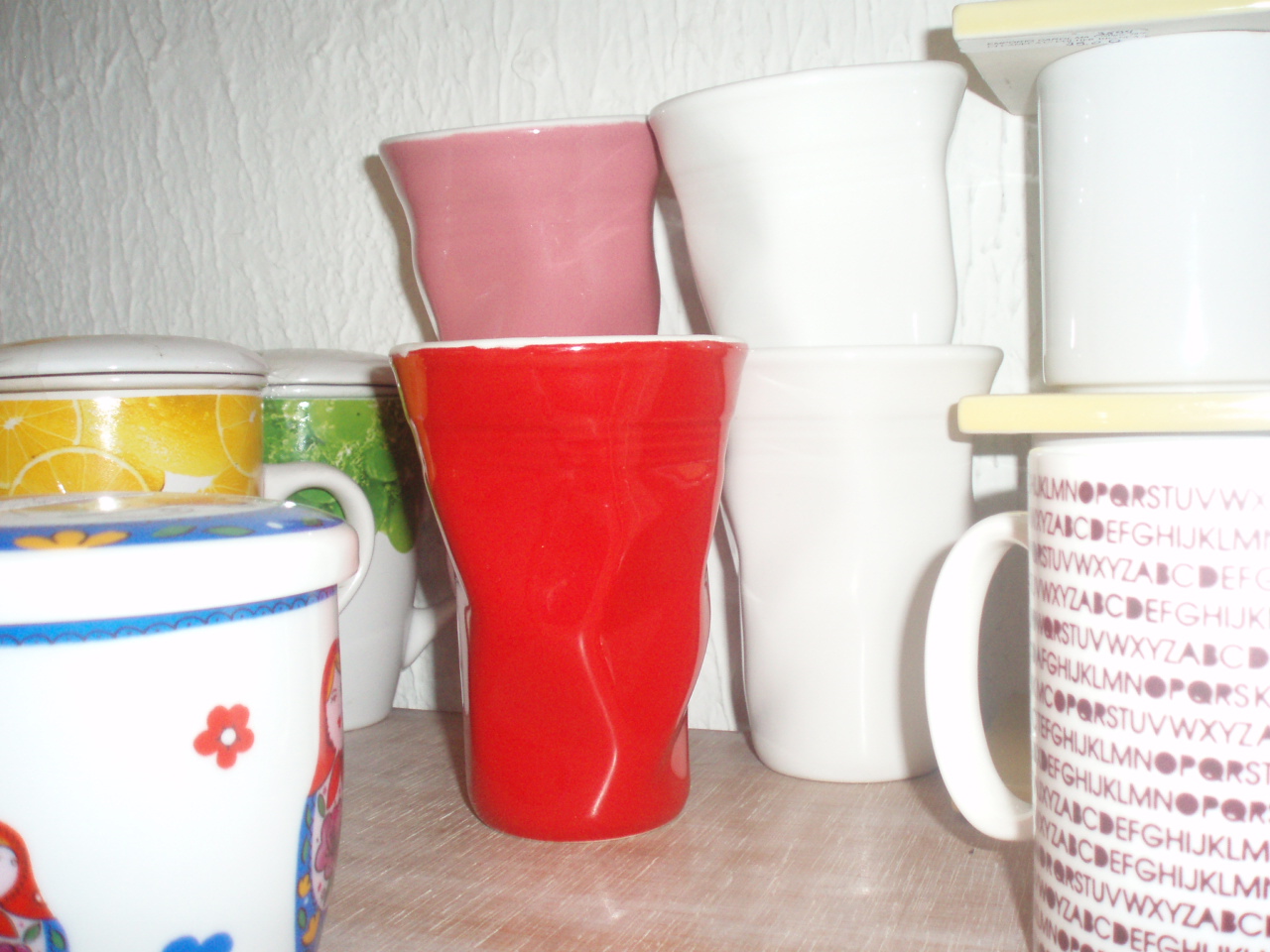This is a detailed photograph showcasing a collection of cups and mugs inside a cupboard against a white, corrugated wall. The cups are displayed on a faded tan brown wooden shelf with white streaks. In the center of the arrangement, there is a standout misshapen red porcelain cup with a white rim and wavy lines towards the bottom. Nestled within this red cup is a pink cup, giving the appearance of being stacked together. To the right of this unusual pair are two stacked white cups, beside which another white cup sits on a small yellow board. Below this arrangement is a white mug adorned with red alphabet letters in a repeating pattern.

On the left side, an array of colorful mugs adds variety: a yellow mug, a green mug, and a white mug decorated with flowers, which also features an image of a girl with red hair and blue dress. At the bottom left corner of the photo, there's a unique white cup with blue markings and Russian nesting dolls depicted around it, showcasing flowers in the center. Behind this, a white mug with a lid displays orange slice images, and another white-lidded mug behind it features grape-like green shapes around the top. This diverse collection of cups and mugs, both plastic and porcelain, provides a charming view of a well-used kitchen storage space.